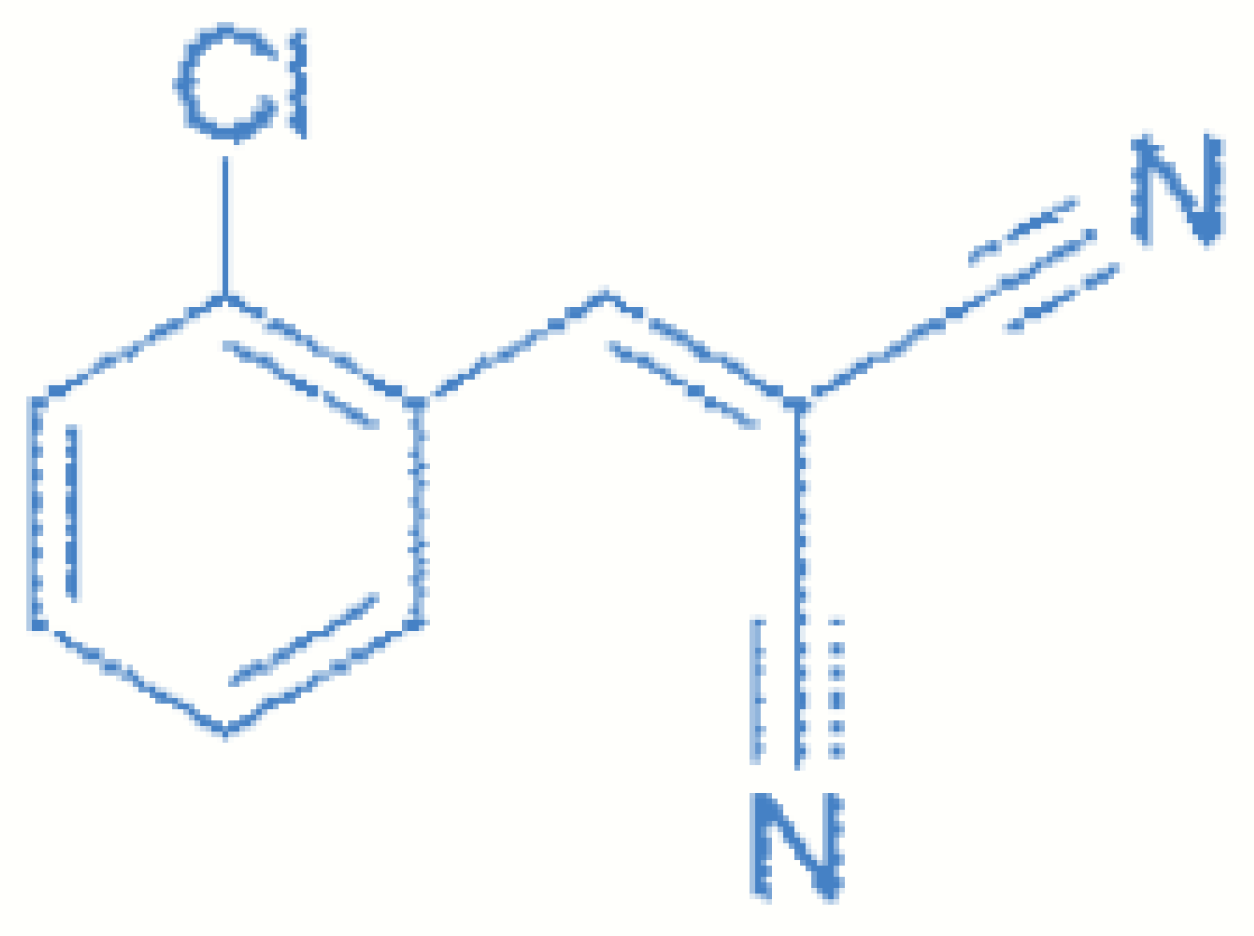The image is a detailed, grainy, and somewhat old-fashioned illustration of a chemical molecule, likely taken from a textbook. The main structure is a hexagonal shape (polygon with six sides) drawn in a light sky blue color against a flat white background. From the top left of the hexagon, there's a line leading to the letters "CL". From two adjacent points of the hexagon, there are lines branching out; the upper line points to a letter "N," and the lower line also points to a letter "N." The overall appearance of the lines and letters is slightly fuzzy, suggesting that the image may have been enlarged, contributing to a blurred effect.